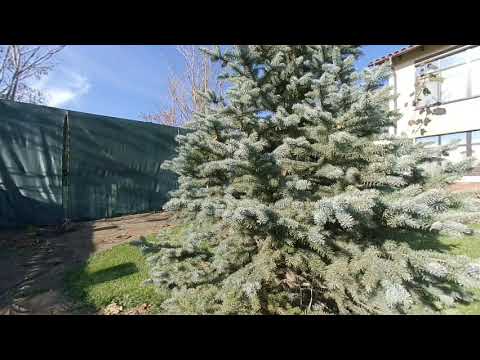This photo captures a large evergreen tree, prominently positioned in the center, showcasing its needle-like leaves in a lightish white-green color, possibly indicating a recent snowfall that has mostly melted. The tree, appearing somewhat untamed and extending beyond the frame, suggests it hasn't been trimmed recently. The setting is a backyard, fenced in by a dark blue or green tarp-covered structure, likely for protection against harsh weather. To the left, the fenced area is visible, and beyond it, a field with patches of grass and dirt. Behind the fence stand several leafless trees that are dusted with snow. On the right, a portion of a two or three-story white house with a light brown, shingled roof can be seen. Above, the sky is blue with a few wispy clouds, completing this serene residential winter scene.